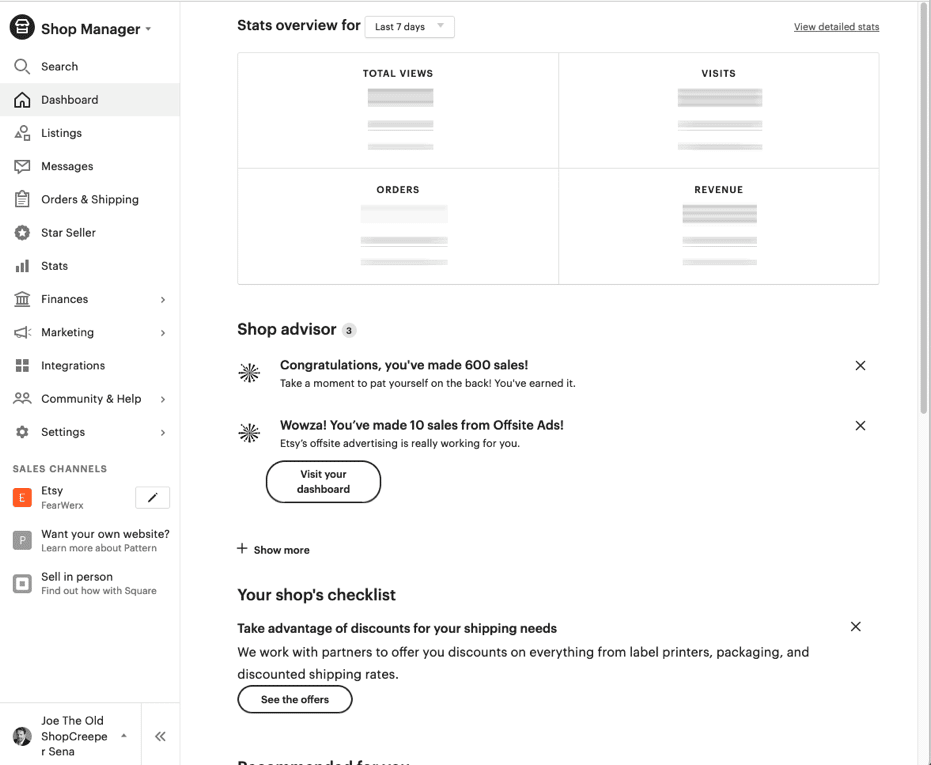The screenshot displays the main interface of a shop management dashboard. On the left-hand side, there is a vertical menu with multiple options in a column. At the top, in bold black font, sits "Shop Manager" accompanied by a logo to its left, indicating it can be clicked for further actions. Below it, in gray font, there are several menu items each paired with an icon: Search, Dashboard, Listings, Messages, Orders & Shipping, Star Seller, State, Finances, Marketing, Integrations, Community & Help, and Settings.

Further down, under the heading "Sales Channels," there are three sections: one for Etsy, marked with its symbol, another for "Want Your Own Website" with info about Pattern, and the last one, "Sell in Person." At the very bottom of the menu, an unconventional label reads "Joe the Old Shop Creep."

On the main part of the screen, current shop statistics are displayed. By default, this section shows data from the last 7 days, but the period can be adjusted. There is a link labeled "View Detailed Stats" on the right side of this section. Key metrics are presented in four stacked squares: Total Views, Visits, Orders, and Revenue, though the specific values for these metrics are currently blanked out.

Towards the bottom of the stats section, a Shop Advisor provides congratulations, highlighting milestones such as reaching 600 total sales and achieving 10 sales via site-wide ads. Various other notifications celebrate the shop's performance and successes.